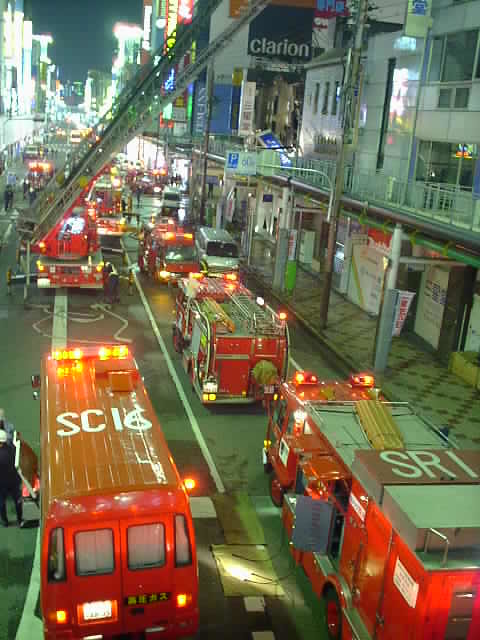The photograph captures a dramatic nighttime scene in a Japanese city, viewed from an elevated position, possibly the first or second floor of a building. The street below is bustling with emergency activity, dominated by a multitude of brightly lit fire trucks and other rescue vehicles. Central in the frame, two fire trucks are prominently visible in the foreground, with their bright orange lights flashing, and additional fire trucks are lined up vertically along the street. The truck in the lower left corner is marked with "SC-16" in white lettering, while the one to the right has "SR-1" displayed on its roof. 

In the background, a ladder truck extends its ladder diagonally from the left towards the upper right, reaching towards a glossy, glassy building, hinting at the urgency of the emergency. Despite the significant rescue presence, no smoke or visible damage is observed on the buildings. Firefighters and bystanders stand around, but the sidewalks remain empty. The scene is illuminated by various city lights and signs, with a noticeable one reading "Clarion" and another indicating "parking".

The street continues into the distance, flanked by apartment buildings with numerous windows and storefronts, but no people can be seen inside. The cityscape’s ambient glow along with the rescue lights creates a vivid yet intense atmosphere capturing the essence of an unfolding emergency.